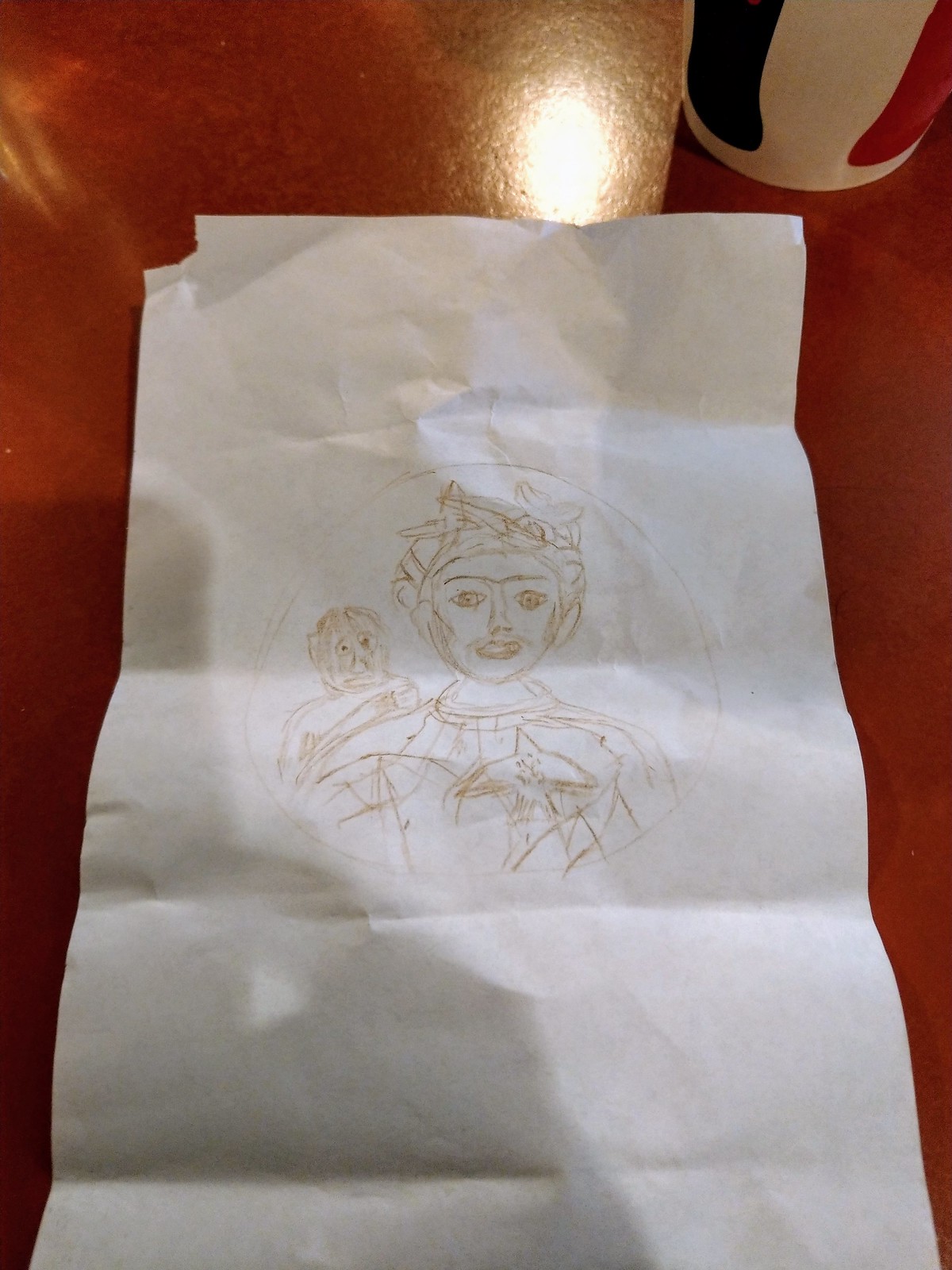In this image, there is a white sheet of paper with faint brown drawing lines sitting atop an orange-colored tabletop, possibly in a restaurant setting. The top of the tabletop reflects light, creating a bright spot at the top of the image. Positioned near the drawing is a white cup adorned with blue and red accents running vertically along its sides. The paper itself, displaying several folds as if it has just been unfolded, features a light brown sketch. The sketch depicts a boy's face with disheveled hair, who appears to be wearing a shirt with a bird-shaped pendant. Positioned behind the boy's shoulder is a monkey figure, adding an intriguing element to the drawing.